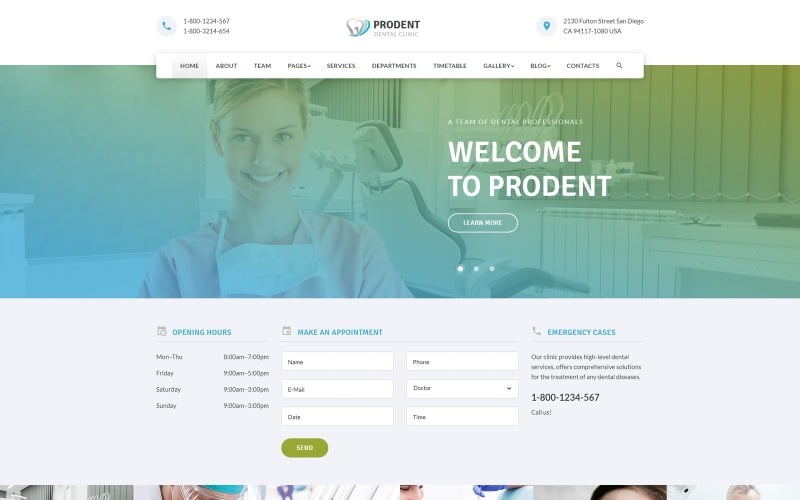In this image of a page, the top left corner features two prominent phone numbers for contact. Centrally located at the top, the business name "Prudent Dental Clinic" is displayed in bold text. On the top right corner, the address is clearly listed as "2130 Fulton Street, San Diego, California, 94117-1080, USA." Below the header, a navigation bar includes links to sections such as Home, About, Team, Mobile, Services, Departments, Timetable, Gallery, Blog, and Contacts. The main visual features a lady smiling with a dental clinic backdrop, enhancing the welcoming message: "Welcome to Prudent Dental Clinic."